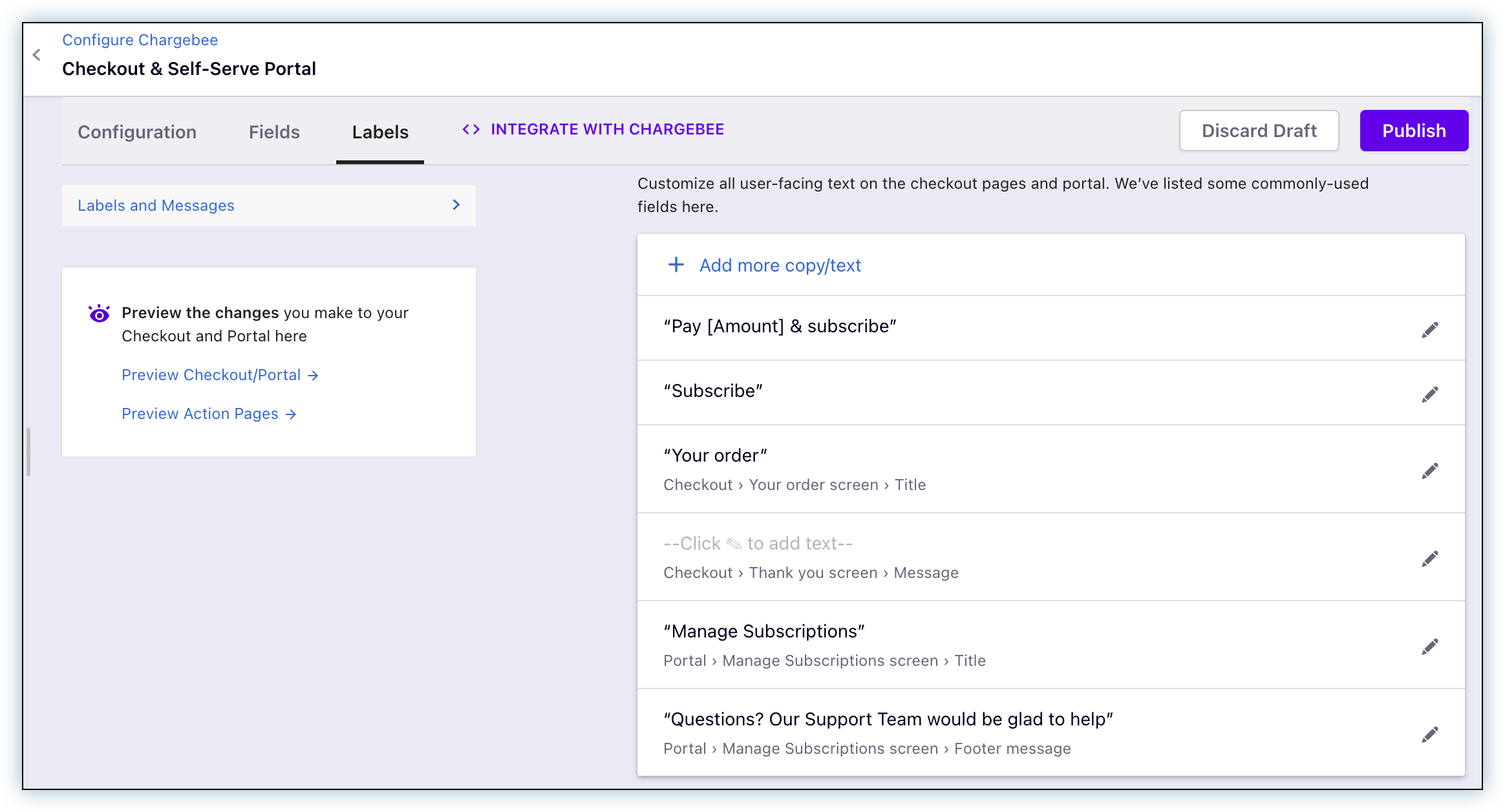The image depicts a screenshot of a user interface from a platform or portal, identified as 'Configure ChargeBEE'. At the top of the screen, the header text reads “Configure ChargeBEE” in bold letters, followed by “Checkout and Self-Serve Portal”.

Just below the header, a series of tabs are displayed horizontally, starting with “Configuration”, followed by “Fields”, and then “Labels”. Additionally, there is an option labeled “Integrate with ChargeBEE” highlighted in purple text. The current active tab in the screenshot is “Labels”.

Within the “Labels” tab, users are presented with various labeling options. The main sections here include “Our Labels” and “Messages”, with additional menus possibly accessible through these sections. Other available options include “Preview the Changes,” “Preview Checkout Portal,” and “Preview Action Pages,” which likely navigate to different sections of the platform for review purposes.

A detailed section beneath these options allows users to add, copy, or edit text. It displays a list of pre-existing labels such as “Pay Amount,” “Subscribe,” “Your Order,” “Manage Subscriptions,” and a customer support message: “Questions? Our support team would be glad to help.”

At the top right corner of the page, there are actionable buttons for “Publish” and “Discard Draft,” enabling users to either save their changes or discard them entirely.